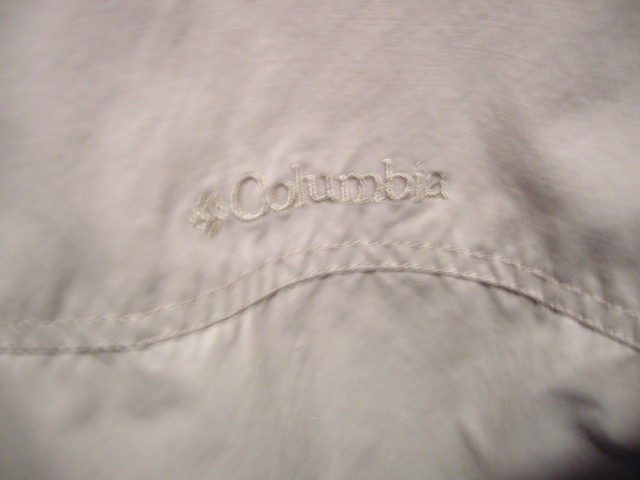This image showcases a close-up view of the back of a Columbia windbreaker jacket. The fabric appears to be a light gray or tan color, bearing the Columbia logo prominently stitched in the same color, giving it a monochromatic look. Directly beneath the logo, a row of zigzag stitches, designed in a triangular pattern, spans horizontally across the fabric, adding a distinct textured detail. This stitching is characteristic of Columbia's windbreaker and canvas jackets. The fabric has a shiny, slightly reflective quality typical of lightweight polyester materials used in such apparel. The image is a bit blurry and out of focus, but it clearly highlights these specific design elements.